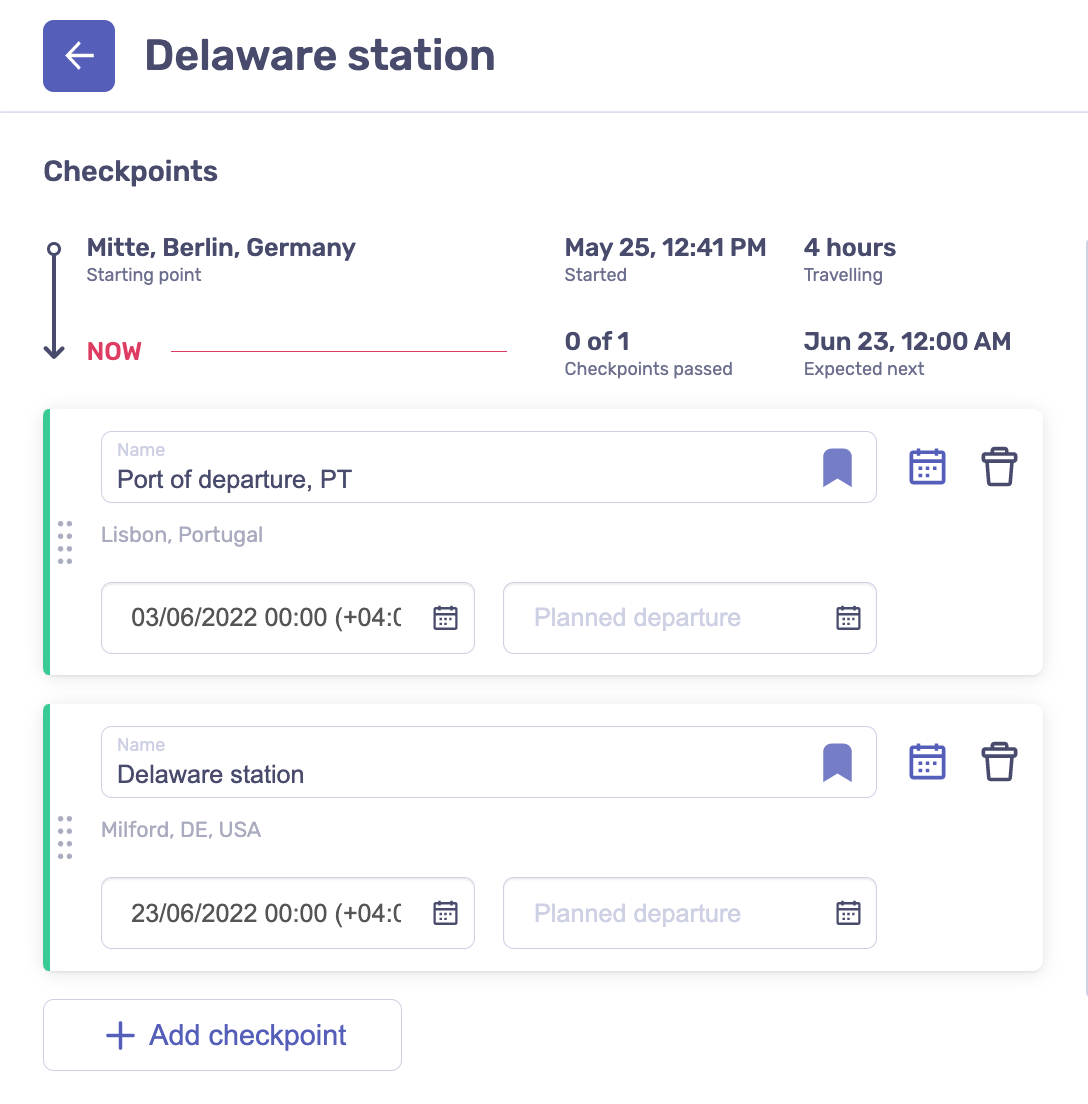This image appears to depict a public transportation schedule interface. At the top, prominently displayed in black letters, is the title "Delaware Station." Directly beneath this header is a section labeled "Checkpoints." Listed checkpoints include MIT in Berlin, Germany, with a travel status that started on May 25th at 12:41 p.m. The trip duration is indicated as four hours, and the current status is shown in red, with a red line next to it, signifying that the travel is currently in progress. It also notes that zero out of one checkpoint has been passed, with the next one expected on June 23rd at 12:00 a.m.

Below this section, there is an entry field for the port of departure, labeled "Port of Departure, PT." Adjacent to this is a time selection box, displaying a date and time as "3-6-2022-0000," indicating midnight. The text next to this box appears to be incomplete or cut off, suggesting it doesn't fully fit within the designated space.

Further down, another name field is visible, labeled "Delaware Station." The accompanying details show "Milford, Delaware, USA," with the planned departure set for "23-6-2022-0000," again indicating midnight. Similar to the previous section, there is text next to this that also seems truncated and doesn't fit the box completely.

Overall, the interface appears to be an organized but somewhat cluttered schedule for various travel checkpoints, detailing both current and future travel plans for different parts of the world.